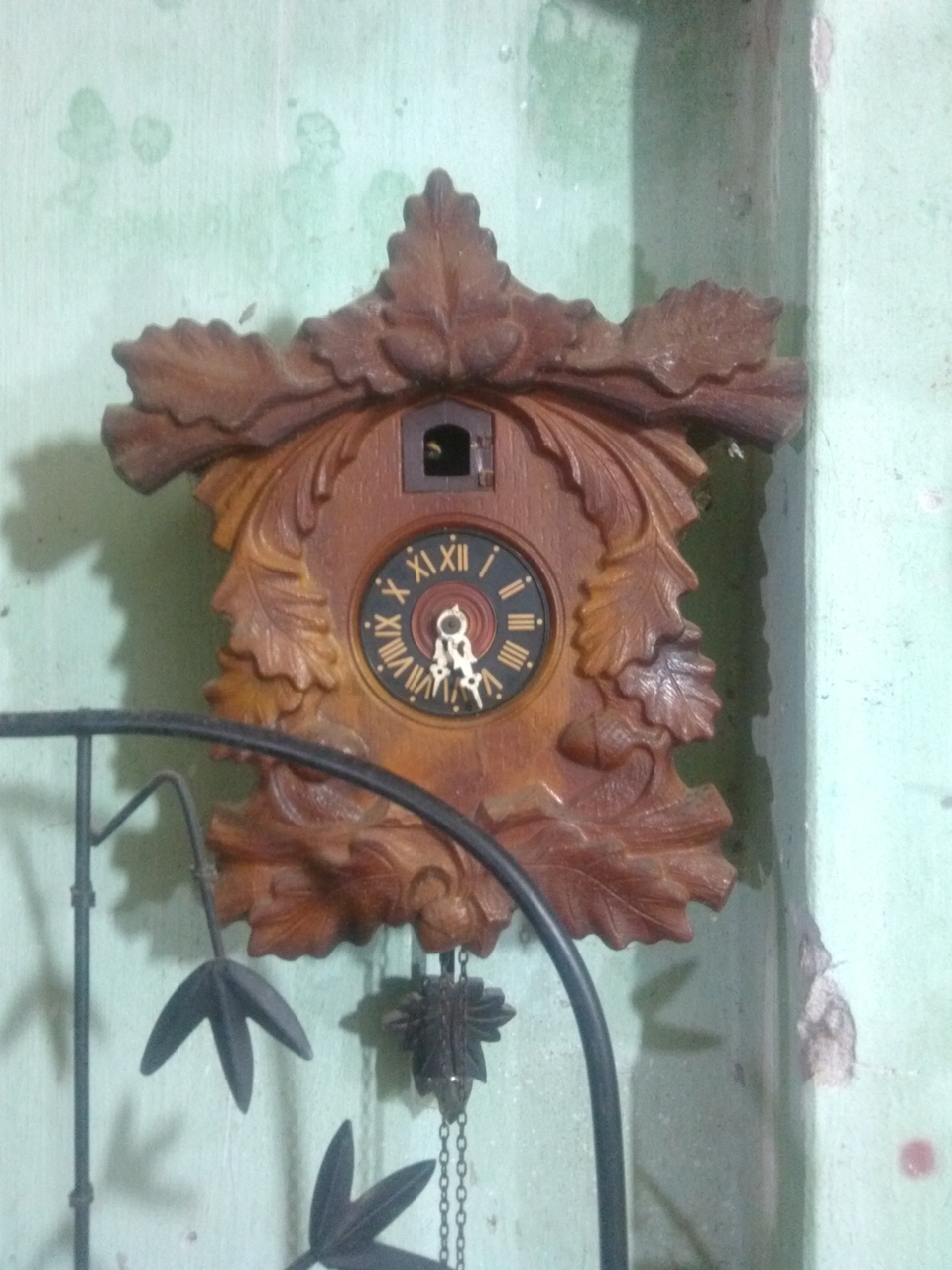The background of the image features a green stone texture, with the right-hand side brightly illuminated in a light blue hue. In the bottom left corner, there are visible elements that resemble plants, branches, and leaves. Mounted on the wall is an ornate cuckoo clock. The clock is heavily adorned with leafy designs at the top, center, and bottom. 

The clock face displays the numbers 1 through 12, each separated by dots. The hands of the clock are positioned between the hours of 6 and 7, suggesting it is slightly past 6 o'clock. At the top of the clock is a small hatch from which the cuckoo bird emerges. Below the clock face, there are weights that regulate the time; winding these weights activates the clock mechanism. 

Overall, the intricate combination of natural elements and the detailed design of the cuckoo clock create a visually captivating scene.